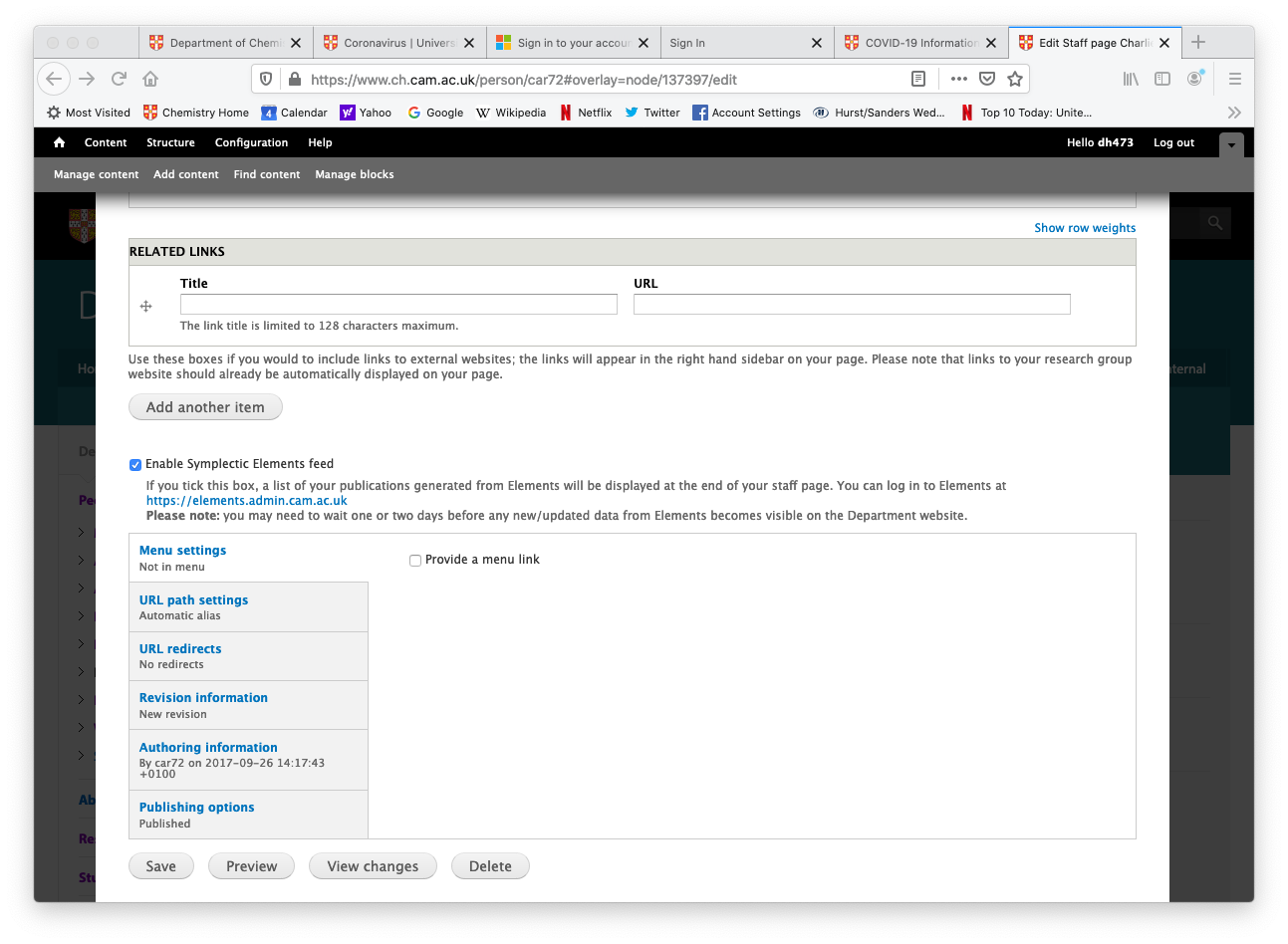This image captures a detailed view of a web browser displaying multiple open tabs at the top, including "Department of Chemicals," "Coronavirus," "Sign-in to Your Account," "Microsoft," "Sign-in," and "COVID-19 Information." The active tab is titled "Edit Staff Page," with the web address visible as "www.ch.cam.ac.uk/person/car72#overlay=node/137397/edit." 

In the main content area of the page, there are several options such as "Manage Content," "Add Content," "Find Content," and an "Image Box." A section labeled "Related Links" is also present, and the checkbox for "Enable Sympletic Elements Feed" is marked as selected. Additionally, there is a vertical menu located on the lower-left side of the screen, suggesting further navigation options.